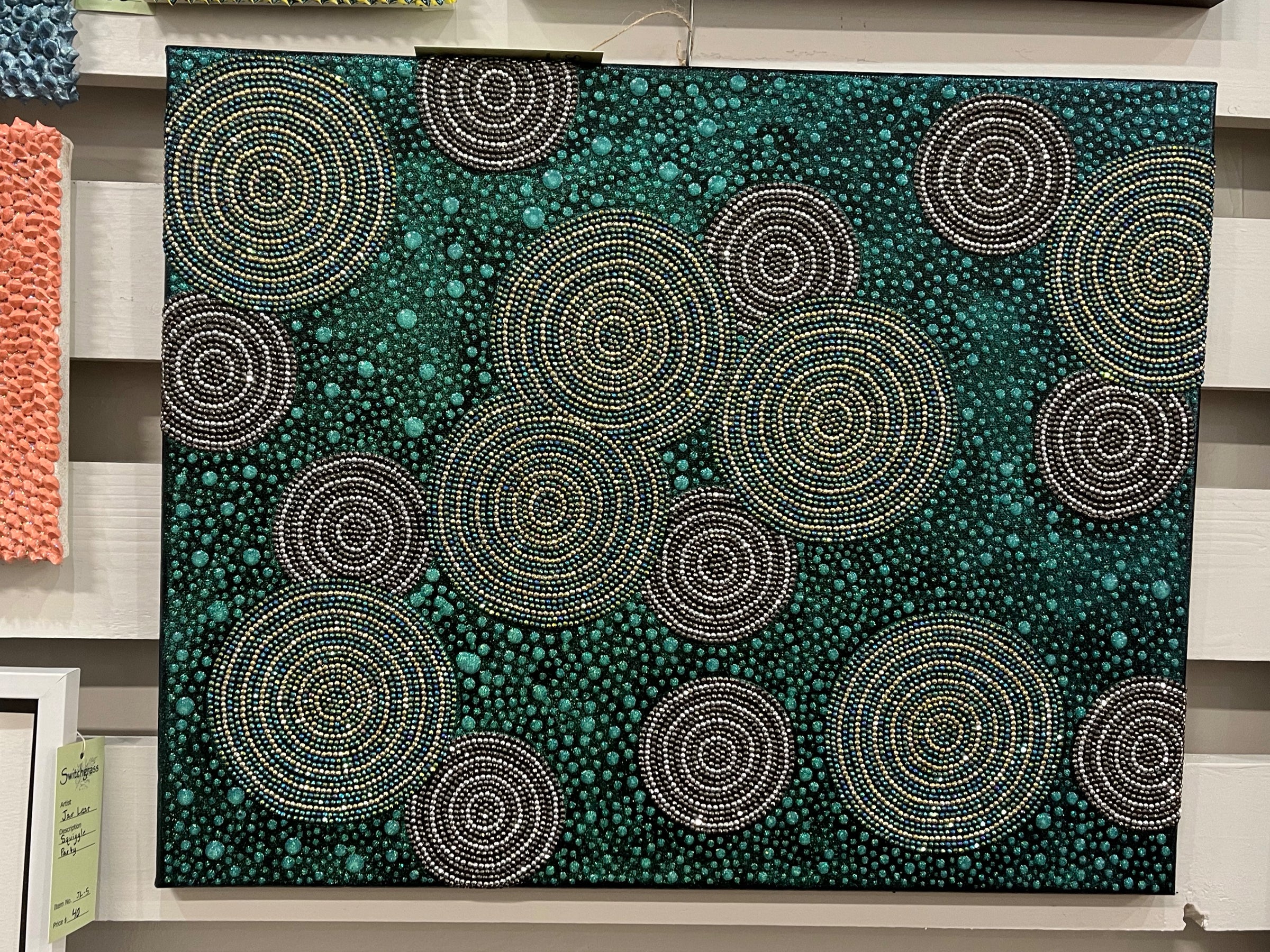This is an intricate art installation photographed in color, showcasing a square mosaic tile piece displayed on a horizontal wooden wall in an art gallery. The centerpiece, a perfectly square tile art, features a complex background of dark green and blue hues with multiple green, white, and yellow circular designs scattered across its surface. There are a total of 17 circles of various sizes, some partial at the edges, creating a playful yet ordered pattern. The circles are arranged across the green and blue backdrop, with some areas appearing to have intricately woven round mats. The mosaic has both smooth and rough textures, enhancing its tactile quality.

In the upper left corner of the art piece, a similar circular and color pattern appears but is only partially visible. To the left of the main subject, there are hints of other art pieces featuring orange and brown circles, suggesting a theme or series. The lower portion of the image reveals a white frame detail, and a tag hanging from the mosaic artwork confirms its curated display in a gallery setting. Additionally, the wooden wall on which it hangs provides a neutral, yet contrasting background, making the vibrant and detailed artwork stand out prominently.